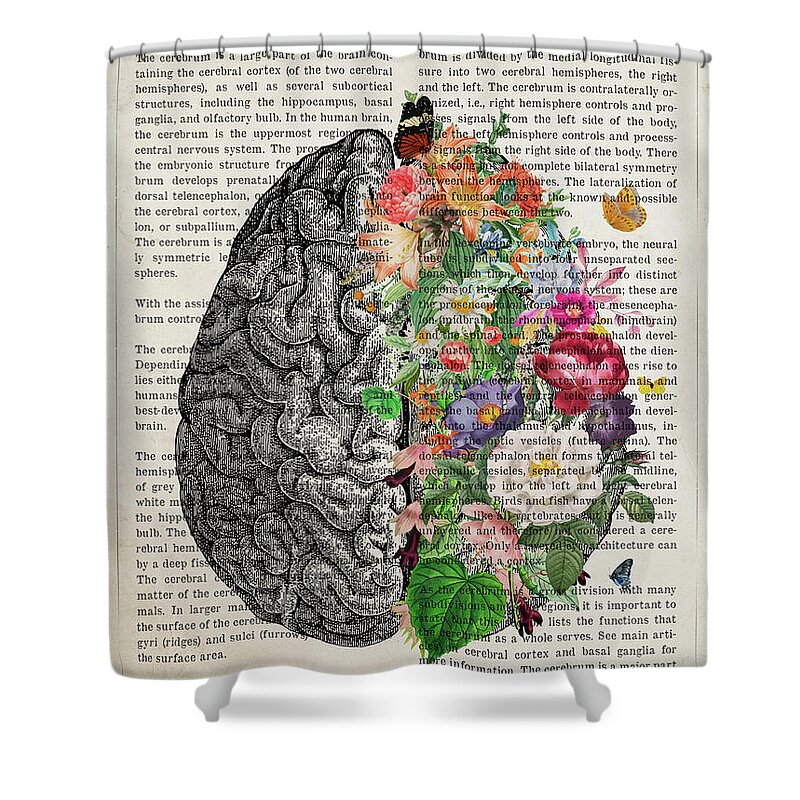This detailed image depicts a shower curtain adorned with an intricate design and suspended from a curved arc shower curtain rod, which provides extra space. The off-white shower curtain is entirely covered in text. Superimposed over this text is a large brain illustration spanning nearly the full length of the curtain. The left hemisphere of the brain is a meticulously detailed black-and-white sketch, reminiscent of a medical textbook illustration. In vivid contrast, the right hemisphere is an imaginative composition of colorful flowers, leaves, butterflies, and other creatures, all arranged to maintain the brain's shape, suggesting the flourishing life and creativity. Only the claw-foot legs of the bathtub are visible beneath the curtain, grounding this surreal visual amalgamation in a bathroom setting.